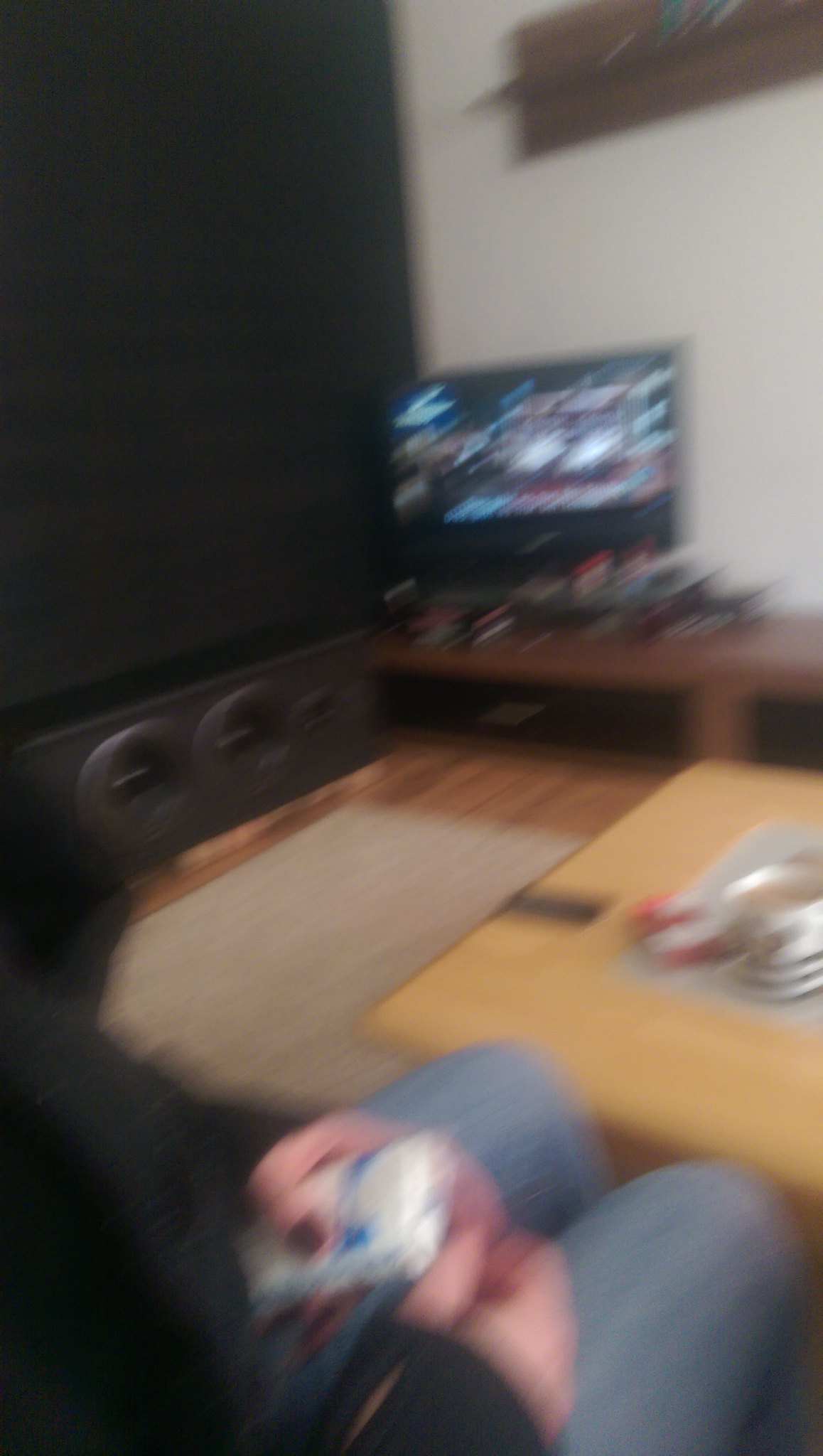This color photograph, though blurry and taken in dim indoor lighting, provides a glimpse into a cozy, possibly living room space. In the foreground at the bottom of the image, a person wearing blue jeans and a dark top is seen holding a rectangular white object with a blue stripe. Their left hand, adorned with dark nail varnish, adds a touch of personality to the scene. This individual stands in front of a wooden table located on the right side of the image. On the table, a cup, likely containing tea or coffee, sits centered on a tray. The cup features black rims and is situated near a red object to its right. A small black rectangle lies on the edge of the table nearby.

Beneath the table, a grey mat partially covers a brown wooden floor. On the left side of the photograph, a large black rectangle, possibly a speaker system, features two knobs at the bottom, adding to the room's ambiance. In the upper middle portion, a television displays a show with multiple colors flashing on the screen, though the specific content is indistinguishable due to the photo's quality. This television rests on a low wooden desk, which houses several black objects underneath. The backdrop consists of a grey wall with a small frame, potentially a photograph or a mirror, peeking out above the television, adding a finishing touch to the cozy room setting.